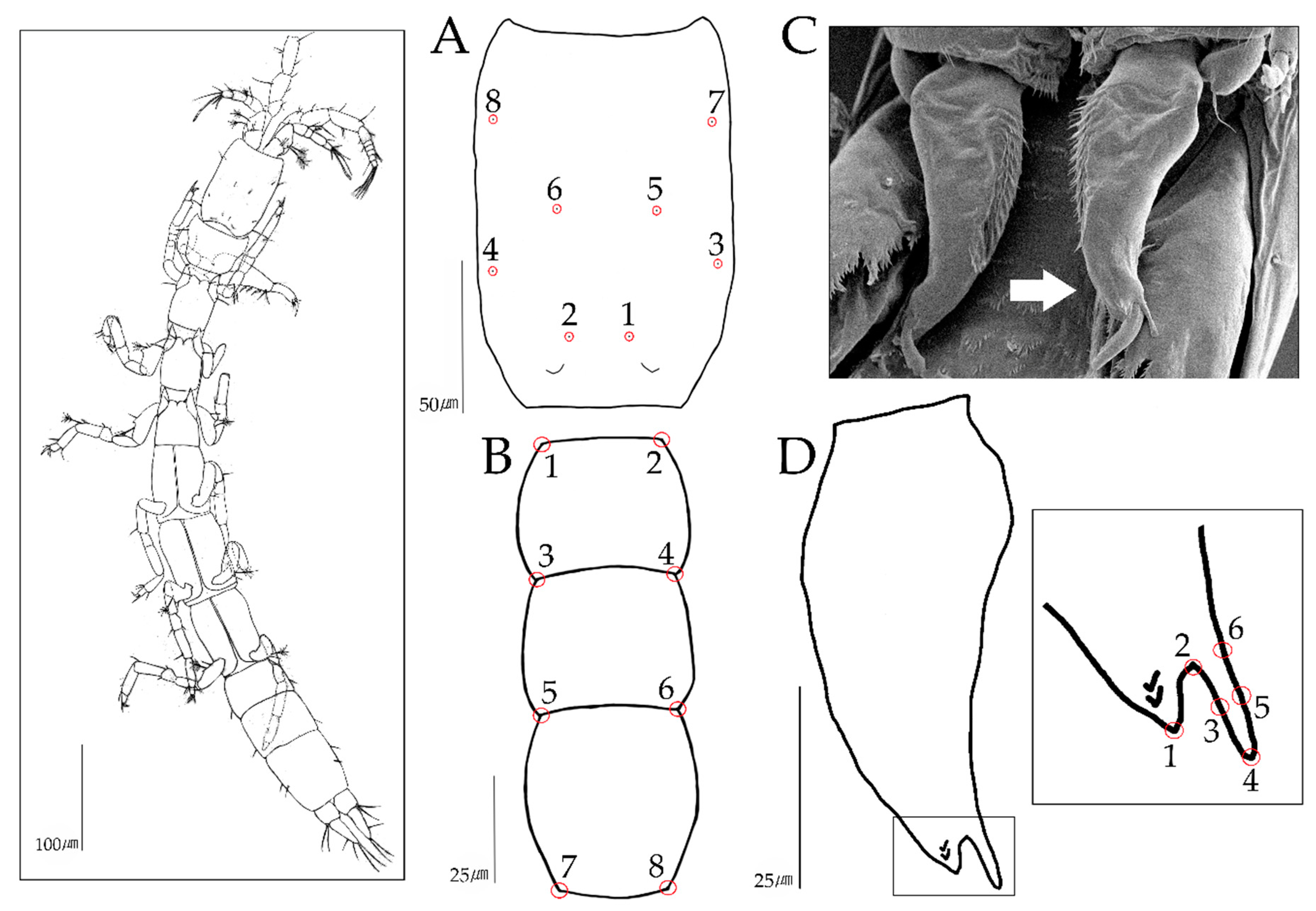This detailed diagram of an insect features four labeled sections (A, B, C, D) and incorporates a total of five distinct images. Positioned on the very left is a full outline showcasing the entire creature. Section A, located in the middle, presents a zoomed-in view of one segment of the insect, clearly numbered from one to eight, offering a close inspection of its anatomical details. Below that, section B mirrors this approach, zooming in on a different body part, also numbered similarly. On the top right, section C provides a live, real image, closely zooming in on the leg of the insect, while section D, just beneath, focuses on yet another part of the creature, possibly the foot, also in a detailed, magnified view. This meticulous representation includes the insect's multiple sets of legs and noticeable antennae, with sections dedicated to dissecting both the middle body parts and the tail, alongside a close-up of the face and its antennae. Overall, the layout and comprehensive labeling evoke a clear, textbook-style presentation.